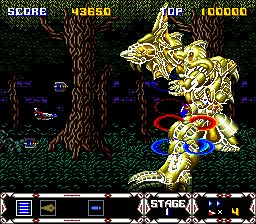This is a screenshot from an old arcade-style video game, likely from the late 1980s or early 1990s, featuring classic pixel art. The scene portrays a forest setting with tall trees characterized by green leaves and brown bark, against a green ground. Amidst the trees, small spaceship-like creatures are floating. Dominating the right side of the screen is a large, gold-colored monster emitting a lightning bolt—reminiscent of a kaiju or dragon figure. The upper left corner displays the score in blue and white, showing 43,650, with "TOP" in capital letters indicating a high score of 100,000. At the lower part of the screen, various character symbols and the stage number, "Stage 1," are visible. Additionally, four remaining lives are indicated in the game's interface. The spaceships are engaging the monster with blue and red lasers, adding to the action-packed atmosphere of this retro gaming experience.